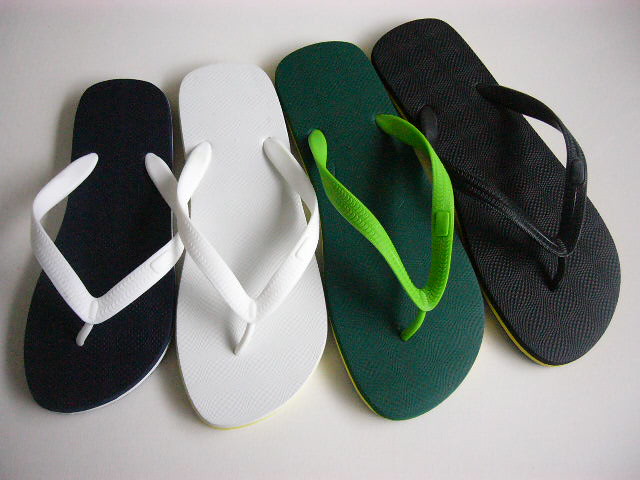This horizontal rectangular photograph features an assortment of four left flip-flops, artistically arranged on a light off-white background with subtle shadowing. Each flip-flop represents a distinct style and color, progressing from smallest on the left to largest on the right. 

Starting from the left, the first flip-flop is black with white plastic straps that form a V, and it has a white trim around the sole. The second flip-flop is entirely white, with matching white straps. The third flip-flop has a deep hunter green footbed paired with light, almost fluorescent lime green straps, and possibly a hint of yellow underneath the green footbed. The final flip-flop is completely black, featuring black straps and aligning towards the bottom right corner of the photo.

These flip-flops exhibit a variety of sizes and are all toe-thong styles, where the strap goes between the big toe and the next toe. The lone appearances of each flip-flop suggest a family assemblage or a curated collection.